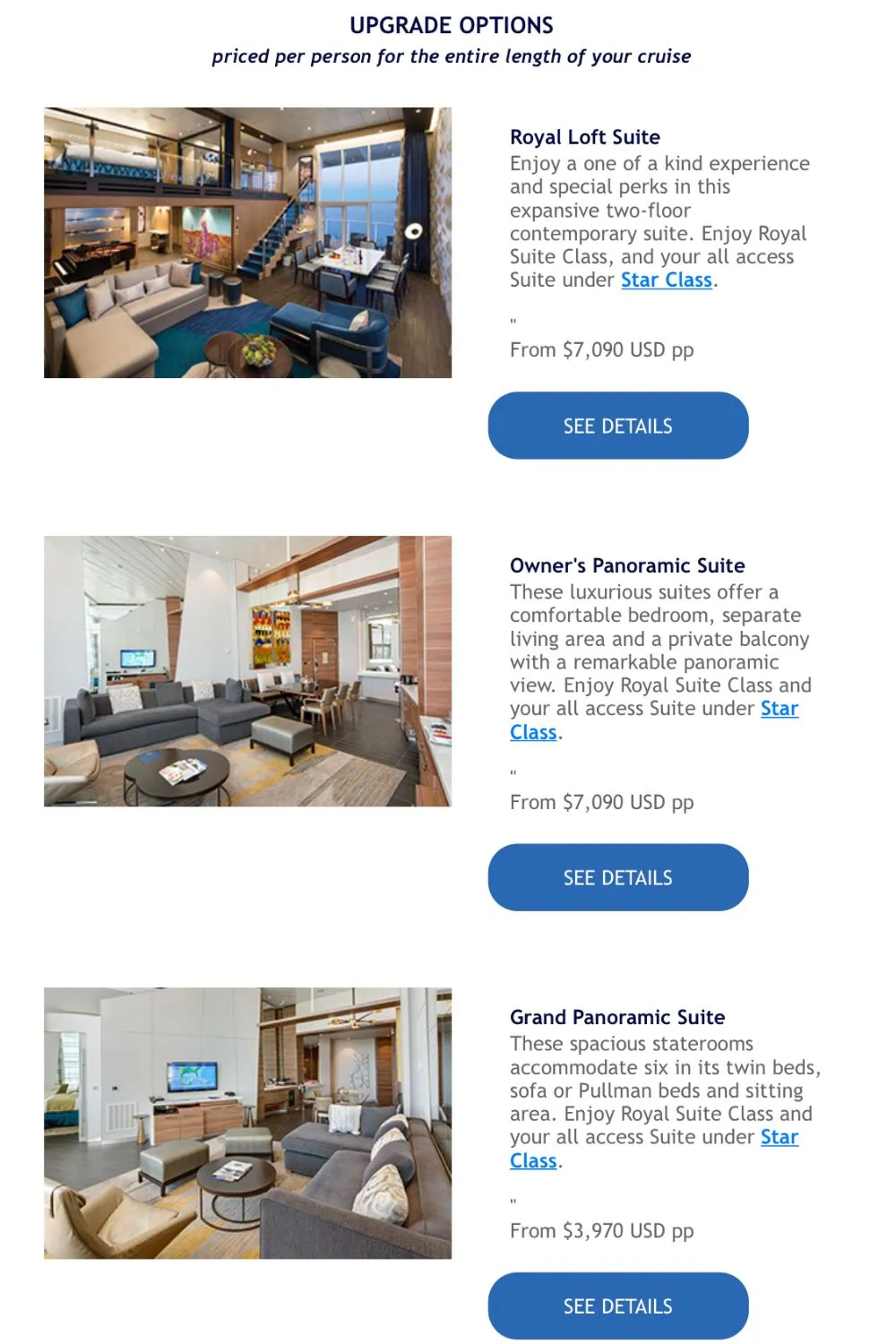The image showcases three luxurious suite options available for cruise passengers who wish to upgrade their accommodations. 

At the top of the image, the text reads: "Upgrade to More Options - Price per person for the entire length of your cruise." 

The first option features the "Royal Loft Suite," described as a unique two-floor contemporary suite offering special perks. Key highlights include access to the Royal Suite Class and the all-access Star Class. The price is listed at $7,090 USD per person. The accompanying image shows a tastefully decorated space with a kitchen, stairs, and blue, gray, and white sofas.

The second option is the "Owner's Panoramic Suite," which offers a convertible bedroom, a separate living area, and a private balcony with stunning panoramic views. Guests enjoy access to the Royal Suite Class and the all-access Star Class. This suite is also priced at $7,090 USD per person. The image depicts a luxurious interior featuring black couches, black tables, and an elegant room setting.

The third option is the "Grand Panoramic Suite," which can accommodate up to six guests. It includes twin beds, a sofa, Parliament beds, and a comfortable sitting area. Guests benefit from the Royal Suite Class and the all-access Star Class, with the price set at $7,090 USD per person. The accompanying image illustrates the spacious layout of the suite.

Each suite description is accompanied by a "Suit Details" button in white text on a blue background. On the left side of each description, there is an image showcasing the interior of the respective suite.

This application allows users to upgrade their cruise accommodation by selecting from these luxurious suite options.